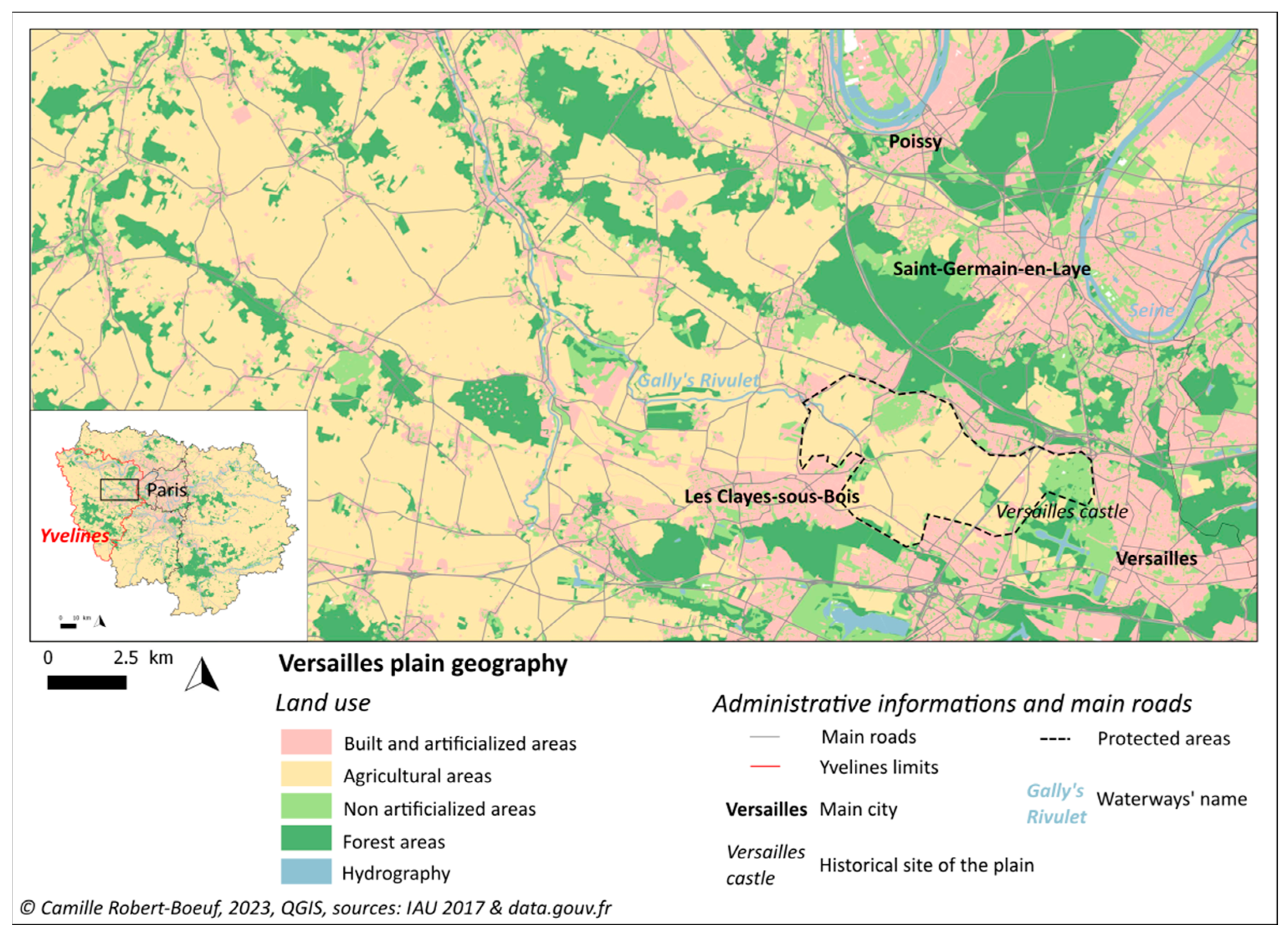The image is a detailed map of the Versailles Plain, segmented into various land uses and geographic features. The top two-thirds of the image display the map itself, which is adorned with shades of yellow, green, pink, and a touch of blue. Notable labeled places in black, including Versailles in the bottom right-hand corner, dot the right side of the map. A white square in the bottom left corner contains a smaller inset map with Paris outlined. 

Below the map, the bottom third comprises a comprehensive key chart explaining the colors and symbols used. On the top left of this area, a black bar indicates a scale from 0 to 2.5 kilometers. Directly below this bar, the key is titled "Versailles Plain Geography Land Use." The key features color-coded categories: a pink bar labeled "Built and Artificialized Areas," a yellow bar for "Agricultural Areas," a light green bar for "Non-Artificialized Areas," a dark green bar for "Forest Areas," and a blue bar for "Hydrography."

Additionally, the bottom section includes headings and smaller text providing administrative information and details about main roads. Small horizontal lines represent various road and administrative data, alongside labels such as "Versailles" in black writing, "Main City" in lighter writing, "Versailles Castle," and the "Historical Site of the Plain."